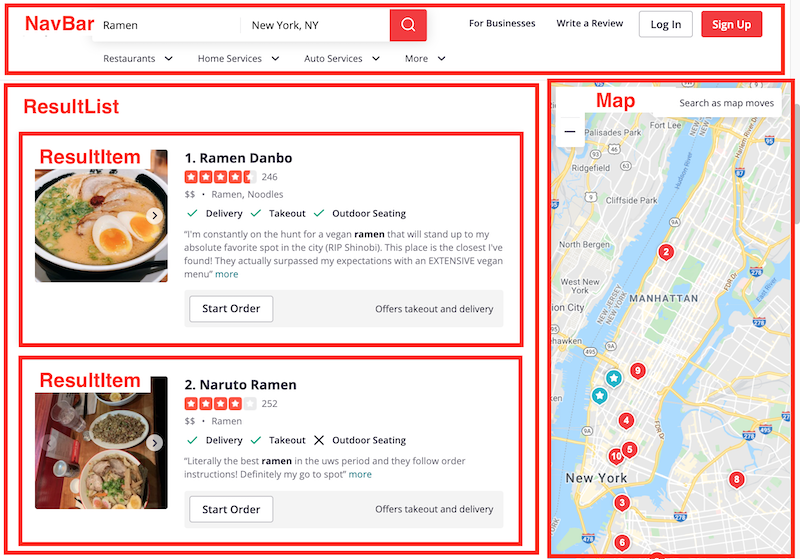The search for ramen places in New York is clearly presented in this food directory interface. At the top of the screen, there's a search bar where users can input their desired food and location, in this case, ramen in New York. Below the search bar, the results are displayed starting with "Ramen Danbo," which has a high rating of 4.5 out of 5 stars. The directory provides additional information such as the cost, indicated by the number of dollar signs (the more dollar signs, the pricier the establishment), and amenities like delivery, takeout, and outdoor seating options. 

A brief review from a previous customer is available for each restaurant, enhancing the decision-making process. There is also an option to start an order directly from the directory, making it convenient for users to either place a takeout or delivery order.

The second listed result is "Niroto Ramen," with a rating of 4 out of 5 stars. Similar to the first listing, it offers options to start an order, along with details on delivery, takeout, and seating availability. In total, there are about 10 ramen restaurants listed, most of which are centrally located in New York City.

The directory enhances convenience by providing a map feature that corresponds with the restaurant listings, showing their exact locations. Users can easily find the restaurant of their choice on the map and use the provided navigation coordinates for directions. This thorough layout ensures a seamless and user-friendly experience for those looking to savor ramen in New York.